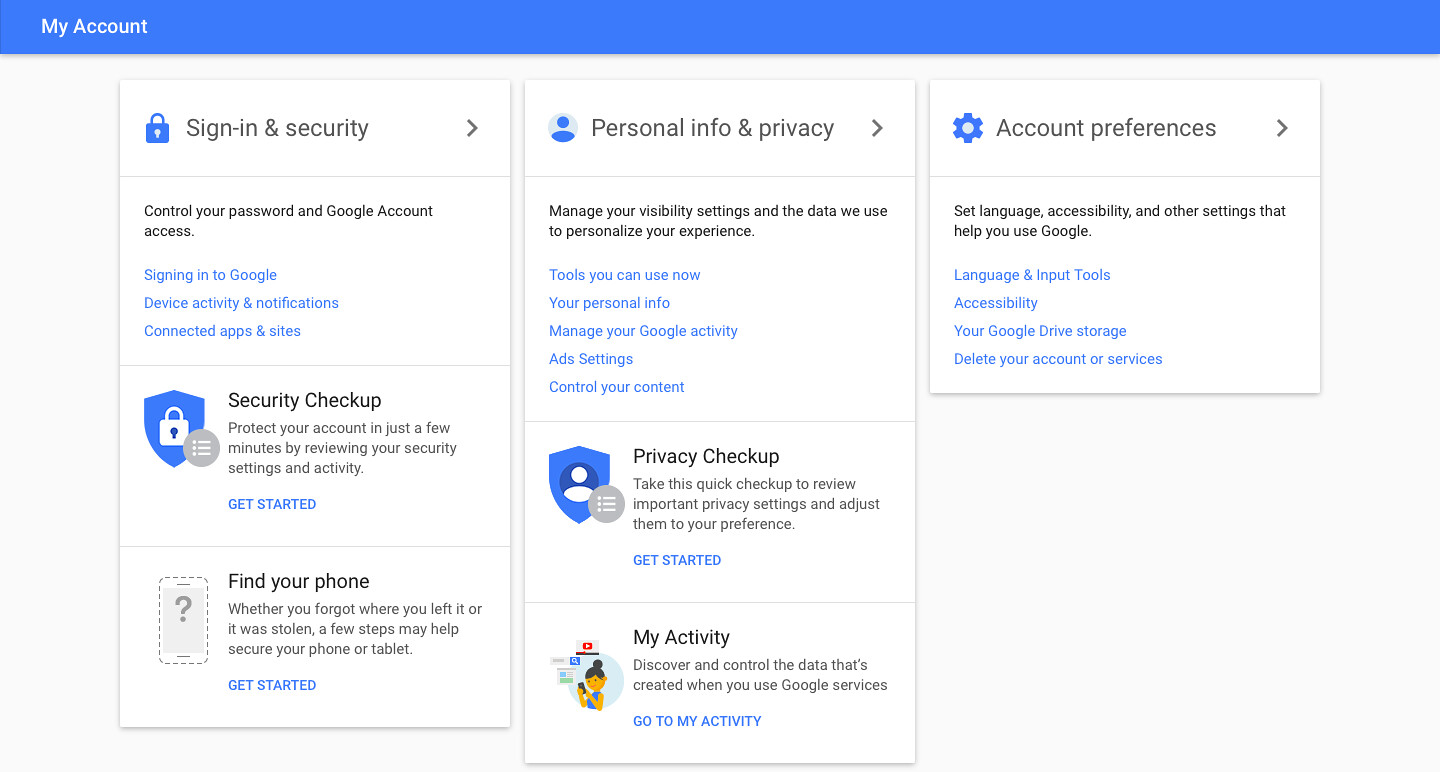In this detailed image, a blue banner spans across the top, prominently displaying "My Account" in white letters on the left side. Below this banner, the background transitions to a light grey color and features three distinct boxes:

1. **Sign-in & Security:** 
   - This box is topped with a blue padlock icon and a grey arrow on the left side.
   - It contains several sections:
     - **Control your password and Google Account access:** Written in black text.
     - **Signing into Google:** Highlighted in blue directly below.
     - **Device activity and notifications:** Listed next.
     - **Connected apps and sites:** Follows below.
   - At the bottom of this box, there are two additional icons:
     - A **Security check-up** icon featuring a badge and padlock.
     - A **Find your phone** icon, showing a phone with a grey interior and a question mark at the center.
     - A search icon for settings, depicted as a circle with three dots and three lines inside.

2. **Personal Info & Privacy:**
   - This section is marked with an image of a person's head and shoulders inside a circle.
   - It includes:
     - **Manage your visibility settings and the data we use to personalize your experience** in black text.
     - Tools you can use now, highlighted in blue, and listed below are:
       - Your personal info.
       - Manage your Google activity.
       - Ad settings.
       - Control your content.
     - At the bottom, a blue badge with a person's face indicates **Privacy check-up**.
     - **My Activity** is mentioned in black text with a cartoonish image of a person looking at their phone displayed below.

3. **Account Preferences:**
   - This box shows a circle with blue ridges on the outside and a central black arrow.
   - It contains:
     - **Settings, set language, accessibility, and other settings that help you use Google** in black text.
     - Further down, highlighted in blue, are:
       - Language and input tools.
       - Accessibility.
       - Your Google Drive storage.
       - Delete your account or services.

Each box is outlined with a delicate light grey line, creating a defined and organized layout for easy navigation.